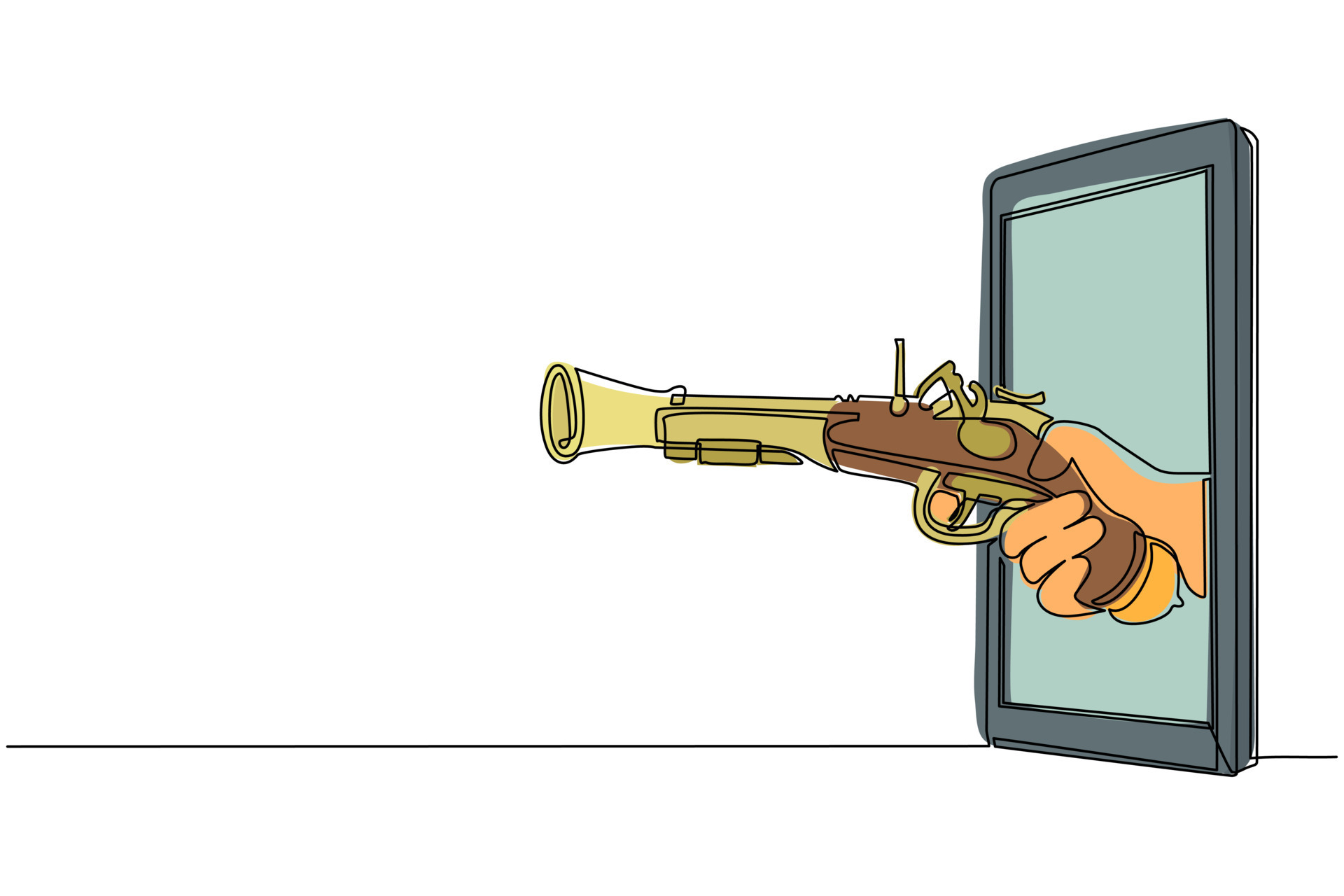This is a detailed and intricate colored artwork set against a stark white background, creating a striking contrast. At the bottom of the composition, a black line suggests a surface or boundary. To the right, a mirror with a gray frame and blue mirrored glass catches the eye. Emerging from the reflective surface is a hand gripping an antique flintlock pistol. The grip of the pistol is rendered in a warm brown hue, while the rest of the firearm showcases a captivating palette of light and dark green tones. Notably, the flintlock mechanism and the trigger are depicted in dark green, providing a subtle yet distinct variation. The barrel of the pistol flares out into a trumpet shape akin to a blunderbuss, adding an element of historical intrigue to the piece.